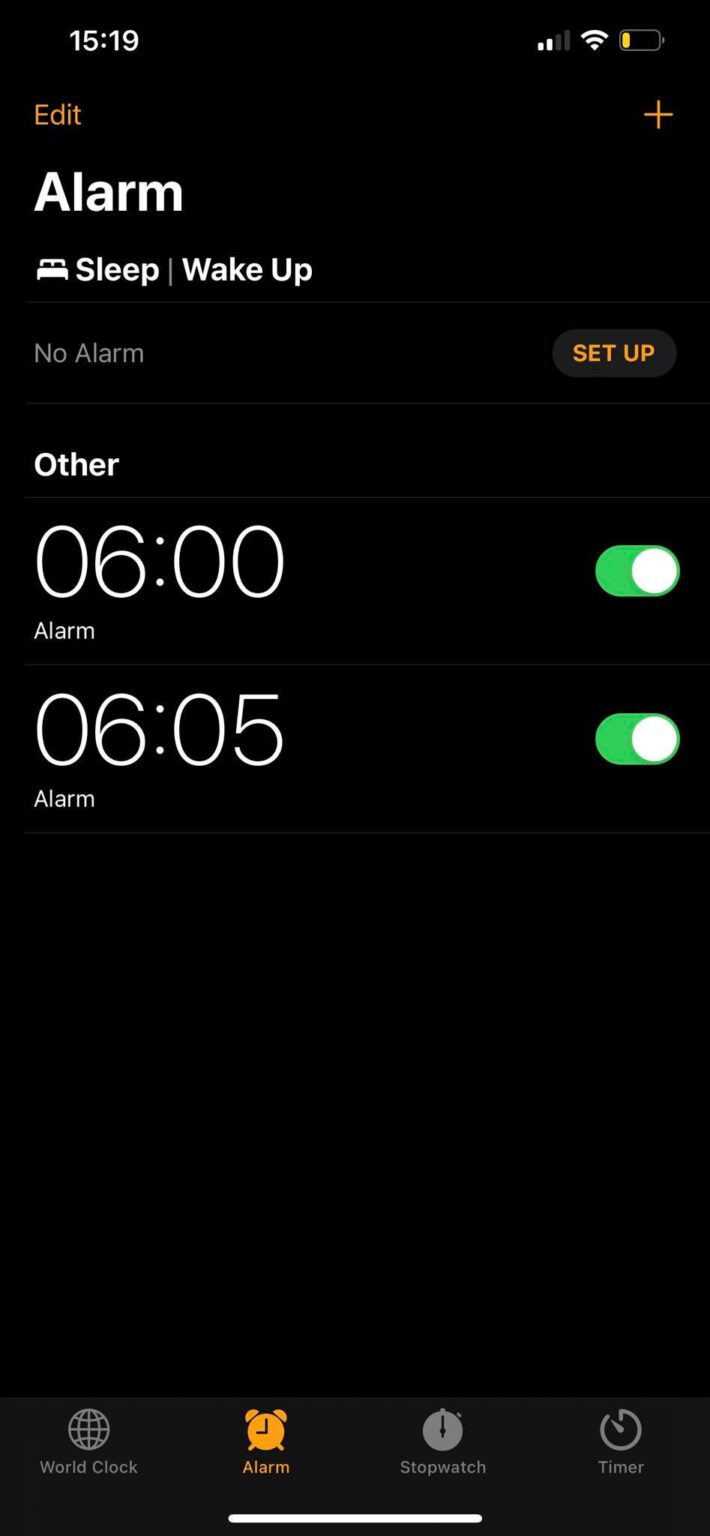Screenshot of a smartphone display with a black background and white text, captured at 15:19 (military time). The device shows two bars for signal strength and Wi-Fi is enabled, with the battery at 20% remaining. On the screen, there is an orange edit button with a plus sign beside it. Below it, the text "Alarm, Sleep and Wake Up" indicates no alarm is currently set, accompanied by an orange "Setup" button. Further down, two alarms are listed: one set for 6:00 AM and another for 6:05 AM, suggesting the user has doubled up the alarms to avoid oversleeping. At the bottom, there's a navigation bar with the "World Clock" and "Alarm" icons highlighted in orange, indicating the screen is currently on the alarm setup page. The options for "Stopwatch" and "Timer" are also visible but not selected.